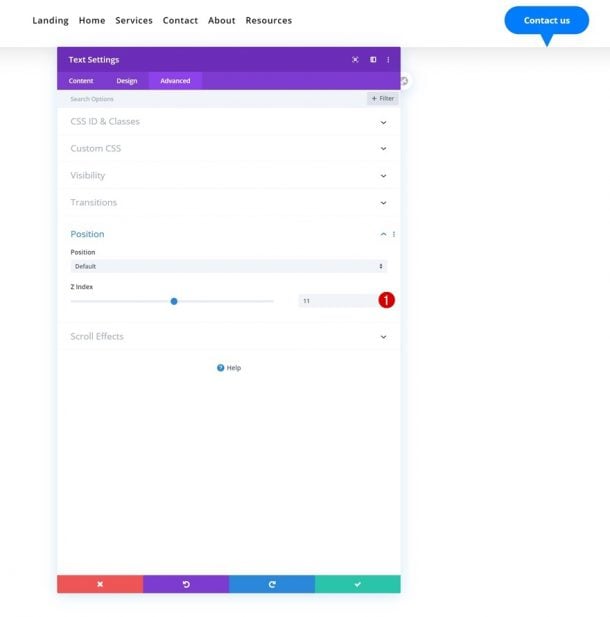**Caption:** 

The image displays a screenshot of an unidentified software platform. The title is absent, suggesting it might have been cropped out. At the very top, several navigation links are visible: "Landing," "Home," "Services," "Contact," "About," and "Resources." On the far right of this navigation bar, a blue speech bubble icon labeled "Contact Us" in white text is prominently displayed.

Central to the screenshot is a settings panel, seemingly a pop-out box, with multiple configuration tabs labeled "Content," "Design," and "Advanced." The "Advanced" tab is currently active, showing various customization options related to web design and styling. These options include fields for "CSS ID and Classes," "Custom CSS," "Visibility," "Transitions," and "Position."

Within the "Position" section, which is expanded, the default position setting is displayed. Below this is a horizontal slider bar for adjusting the z-index. The slider button is positioned in the middle of this bar, indicating a numerical value of 11 on the right side. The overall interface suggests a comprehensive tool for web design or content management.